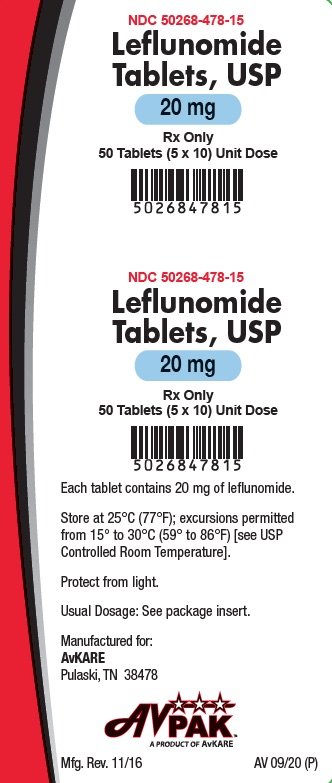A detailed photograph of a pharmaceutical prescription label is presented. The label is primarily white and structured within a vertical rectangle. Along the left edge, there is a sequence of curved bars: an orange bar followed by a black bar and then a gray bar, all curving towards the upper right and lower right sides.

At the top center of the label, "NDC 50268-478-15" is prominently displayed in red letters. Below this, "Leflunomide Tablets USP" is written in bold black lettering. Directly beneath, a blue oval button is visible with bold black text stating "20 milligrams." Following this, it specifies "RX only," "50 tablets," and "(5 x 10)" in black text.

On the right side, the label features a UPC code. Repeating the label information beneath the UPC code, it states: "Each tablet contains 20 milligrams of Leflunomide," followed by storage directions recommending a cool area and protection from light. The usual dosage instructions refer users to the package insert.

At the bottom of the label, it mentions the manufacturer details: "Manufactured for Avcare, Pulaski, Tennessee 38478," accompanied by the AVPAC logo, which includes three stars. Additional details include the manufacturing revision date "11/16" and the code "AV09/20 (P)."